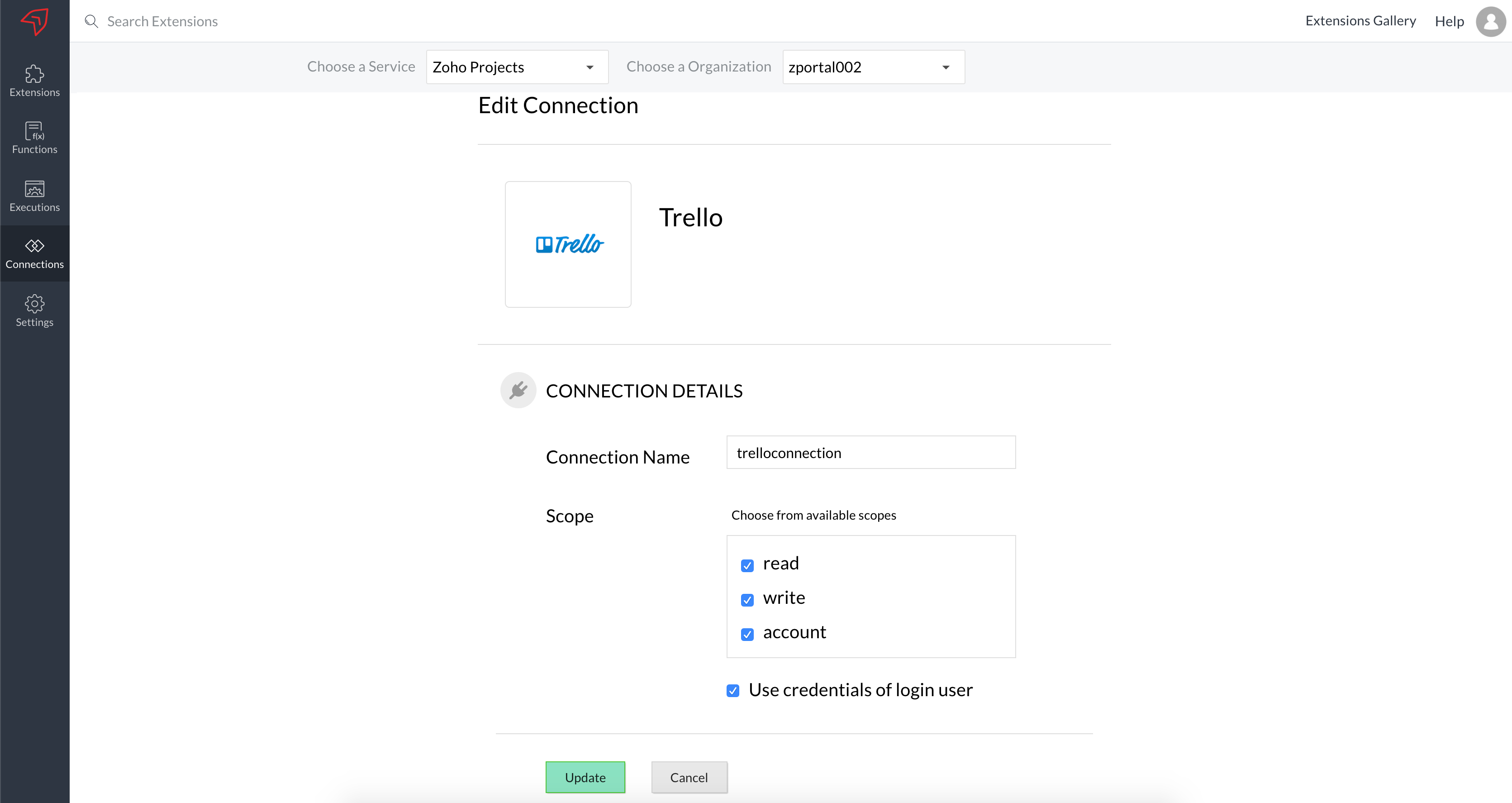The image displays a webpage interface, likely from a platform called Trello or a similar project management tool. The webpage features a black vertical sidebar on the left side, extending from the top to the bottom. At the top of this sidebar is a small red arrow button. Below this button, there are several icons representing different sections: extensions, functions, executions, connections, and settings.

Just beneath these icons, there is a search field labeled "Search extensions," followed by a dropdown menu named "Choose a service," which currently shows "Zoho Projects." Another dropdown menu below this one is labeled "Choose an organization" and displays "zPortal002." The option "Edit connection" appears right after these dropdown menus.

The main section of the page is focused on a connection to Trello. A box with the word "Trello" in blue text appears, accompanied by "Trello" in black letters next to it. Below this, the section titled "Connection details" includes a gray plug icon.

Further down, the interface asks for a connection name, which is set to "Trello connection." Below this, it displays "Scope, choose from available scopes" with multiple checkboxes. The options "Read," "Write," and "Account" are all selected, indicated by blue boxes and check marks.

Finally, the page offers additional options to "Use credentials of login user." At the bottom, there are two buttons: a green "Update" button and a gray "Cancel" button.